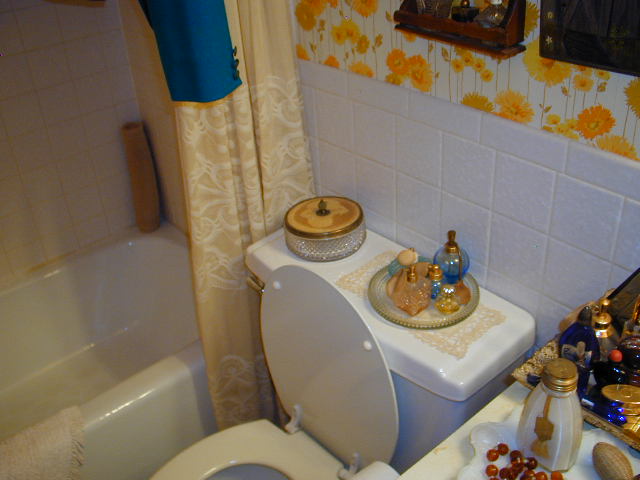This image captures a quaint and detailed segment of a bathroom with several notable features. Dominating the center is the rear section of a light almond-colored toilet, which serves as a display surface for two distinct items. On the left sits a clear glass container embellished with a brownish covering and an ornate handle. This handle is a light orangish-beige with subtle darker brown accents, including a rim in a darker shade. To the right of the container is an off-white lace doily topped with a decorative clear plate that has a scalloped edge tinged with off-white or beige hues. Arranged on this plate are several elegant perfume bottles: a large bluish one with a clear glass top and brass cap, possibly adorned with a tassel; a smaller light blue bottle with a puff; a pinkish bottle with a brass top in the forefront; another smaller bluish one with a brass top; and a yellowish bottle with a silvery-looking top.

Behind the toilet, the wall features a blend of white square tiles edged with rectangular tiles transitioning into wallpaper adorned with light yellowish-orange flowers. Above this, a dark brown wooden shelf holds various indistinct bottles. To the right of this shelf's edge is a dark wooden cabinet, with visible fasteners showing as yellowish round areas.

The right side of the toilet is adjacent to an off-white vanity adorned with textures. Atop the vanity, a golden and blue tray hosts several bottles, including a blue one, a clear one with a brass top, and another slender bottle. Below this tray is a glass jar capped with a wooden cork and a brown tassel, filled with what appears to be a white substance, possibly hand soap. Additionally, there's an obscure oval object and some red beads nearby.

To the left of the toilet sits a bathtub in a matching light almond hue, with an off-white cream-colored bath mat draped over its edge. A shower curtain with a light beige fabric and an off-white design adorns the bathtub’s front, coupled with a blue fabric trimmed with gold. Inside the tub, the walls are decorated with cream-colored square tiles, and in one corner rests a long, cylindrical brown object.

Overall, the image encapsulates a richly decorated and cozy bathroom space with intricate detailing in every corner.